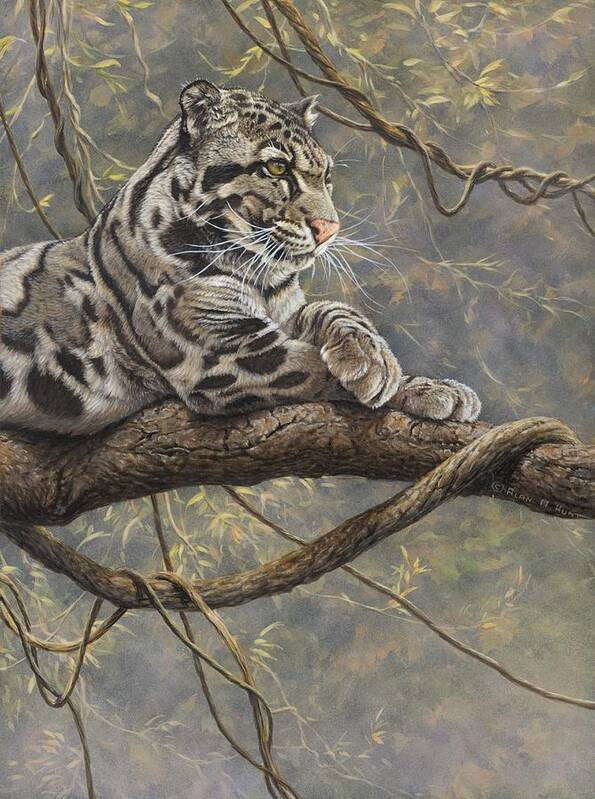The image is a lifelike drawing, copyrighted by Alan Hunt, of a big cat perched on a tree limb in a lush jungle environment. The scene is predominantly green from the dense vegetation, with shrubs and vines hanging around the cat. The cat, which could be a snow leopard or possibly a juvenile leopard, has a grayish-white coat adorned with black spots and thick fur. It is reclined on a thick brown tree branch, gazing off to the right, showing a profile of its face with visible nose and whiskers. The front paws are crossed and the ears are perked up, adding to its alert appearance. The background features various shades of green livery and some faint ground details in browns and greens, making the tree appear quite high.